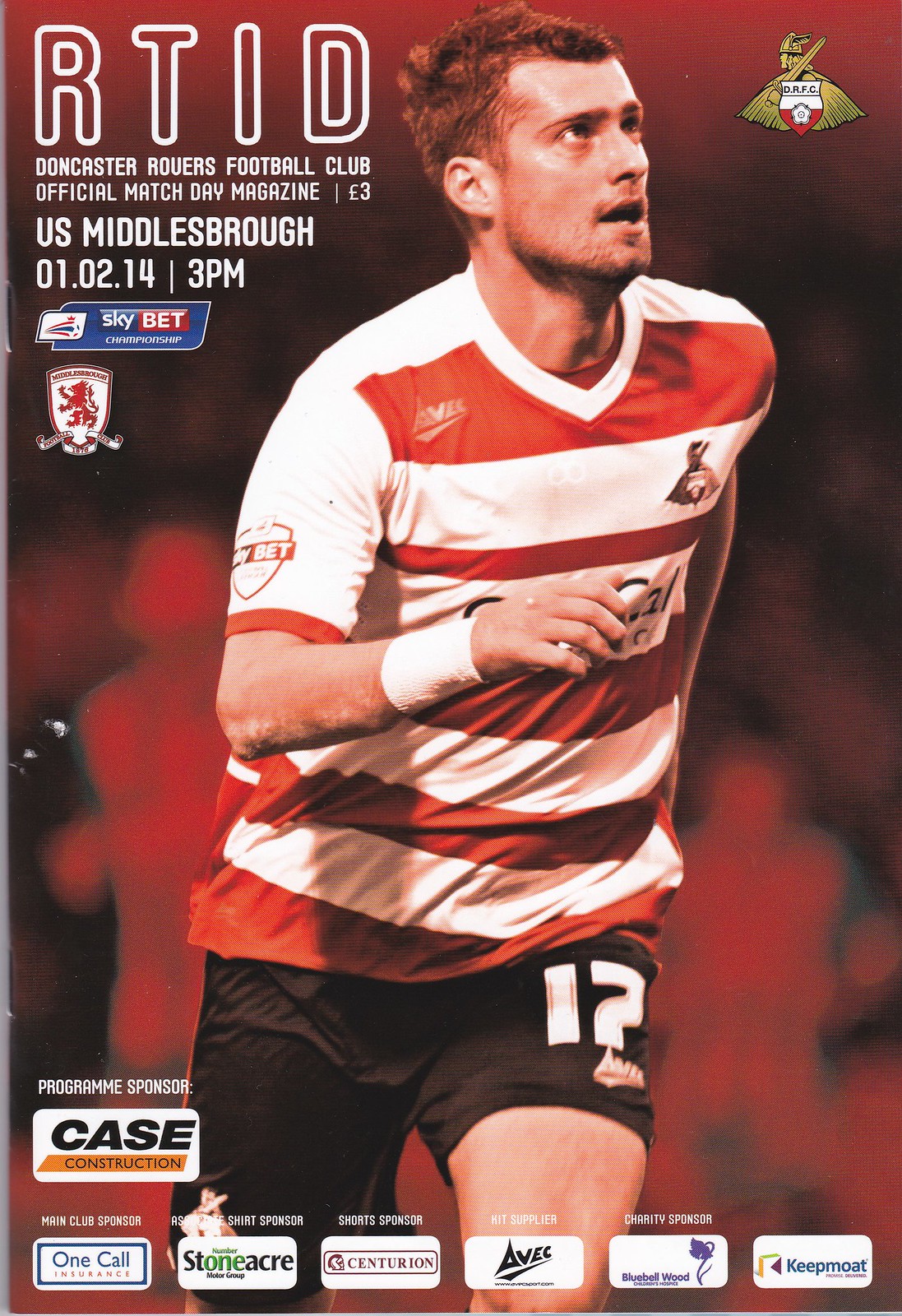The image is of the cover of Doncaster Rovers Football Club's Official Match Day Magazine with a red and black background. In the upper left-hand corner, the magazine title "R.T.I.D." is written in red outlined in white, beneath which it says "Doncaster Rovers Football Club Official Match Day Magazine". Below, the text "U.S. Middlesboro, 01.02.14, 3PM" is displayed, followed by "Skybet". In the lower left-hand corner, "Program Sponsor, Case Construction" is written above several advertisements, including "One Call, Stoneacre, Centurion, AVEC, Bluebell Wood, and Keepmoate." Centrally featured is a player with short brown hair wearing a red and white horizontal striped jersey, black athletic shorts with either the number 17 or 12, and a white wrist strap, presumably a football (soccer) player. The upper right-hand corner has a gold emblem, likely the team's symbol.